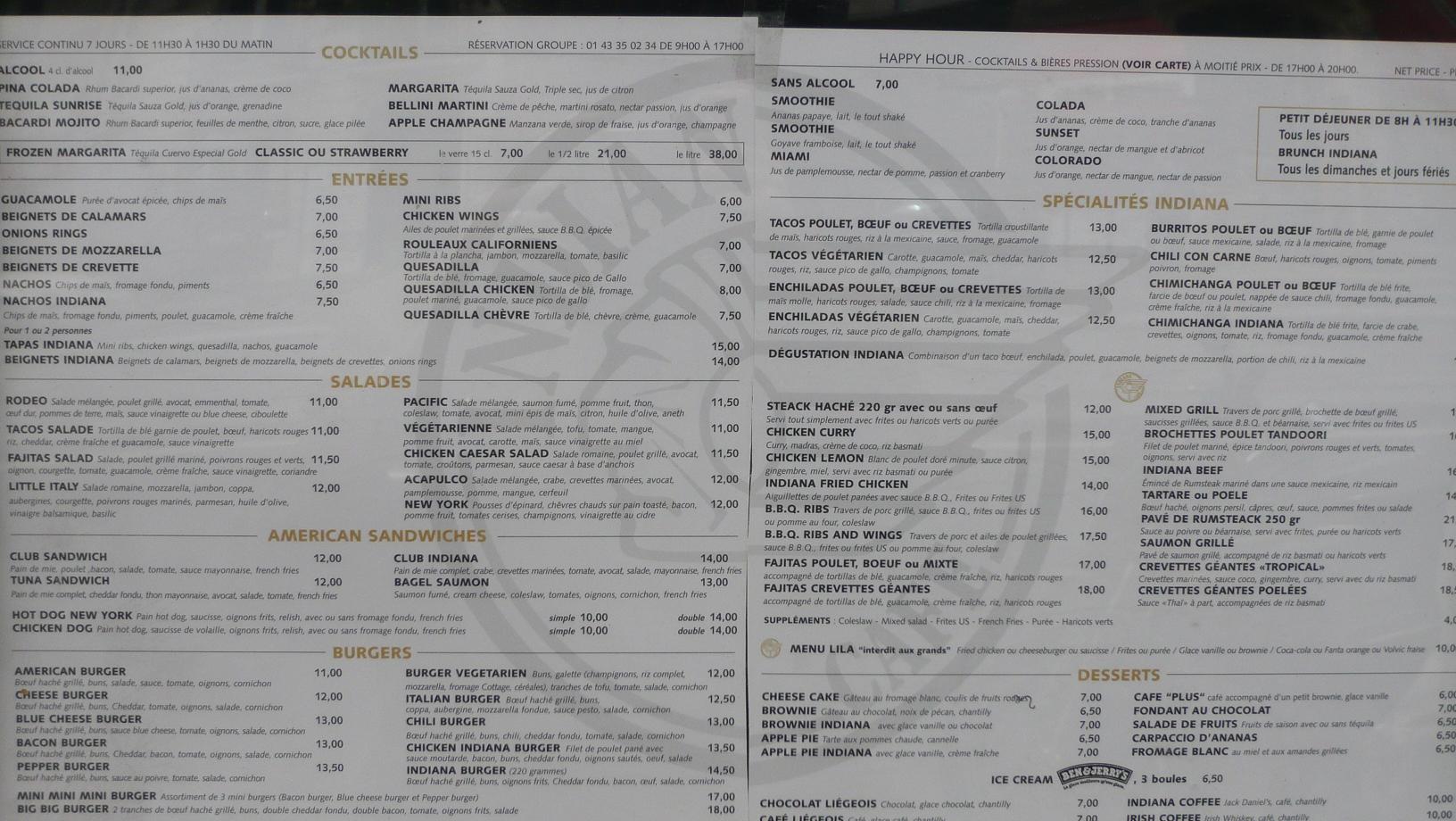This image captures a neatly organized menu written primarily in French, with some English interspersed. The menu is structured in well-defined columns, each with corresponding prices listed. At the top of the menu, there is a reservation contact number: "Réservation Groupe: 01 43 35 02 34 de 9h00." The section headers are highlighted in yellow for easy navigation. These headers include "Cocktails," "Entrées," "Salades," "American Sandwiches," "Burgers," "Spécialités Indiana," and "Desserts." Despite the primary language being French, some dessert items are listed in English, such as "Cheesecake," "Brownie," "Brownie Indiana," "Apple Pie," and "Apple Pie Indiana." The menu offers a variety of dishes and is visually appealing, with an orderly layout that facilitates easy reading.